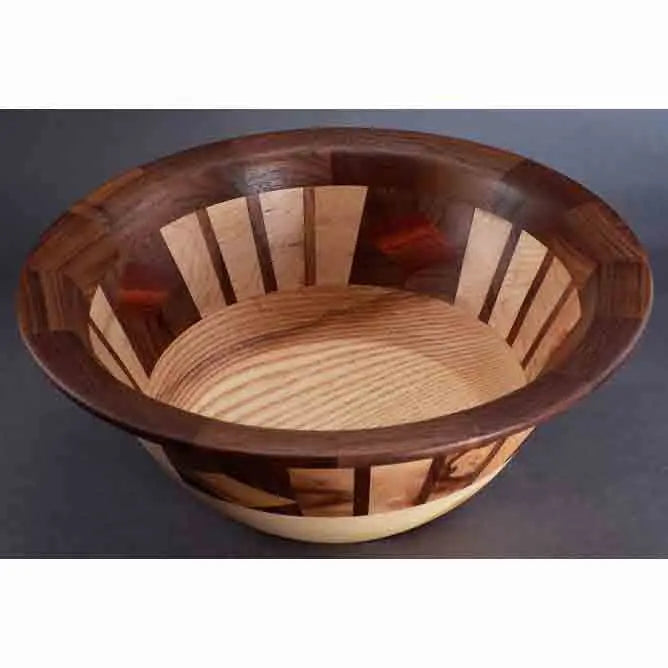This is a beautifully handcrafted wooden bowl, captured in a detailed photograph taken from above at a slight angle. The bowl showcases a striking contrast of wood hues, featuring both light pine and dark mahogany stains. The alternating vertical strips of narrow mahogany and broader pine create a harmonious, rhythmic pattern along the sides. Larger sections of dark mahogany intersperse this pattern, adding a dynamic visual interest to the design. The entire rim of the bowl, which is fluted, is uniformly stained in a deep mahogany, providing a rich, dark contrast to the lighter interior base, which is made from a pale pine wood with visible, lovely grain patterns. The background of the image, a dark gray surface, subtly complements the bowl's rich textures and wood tones, making the craftsmanship stand out distinctly.